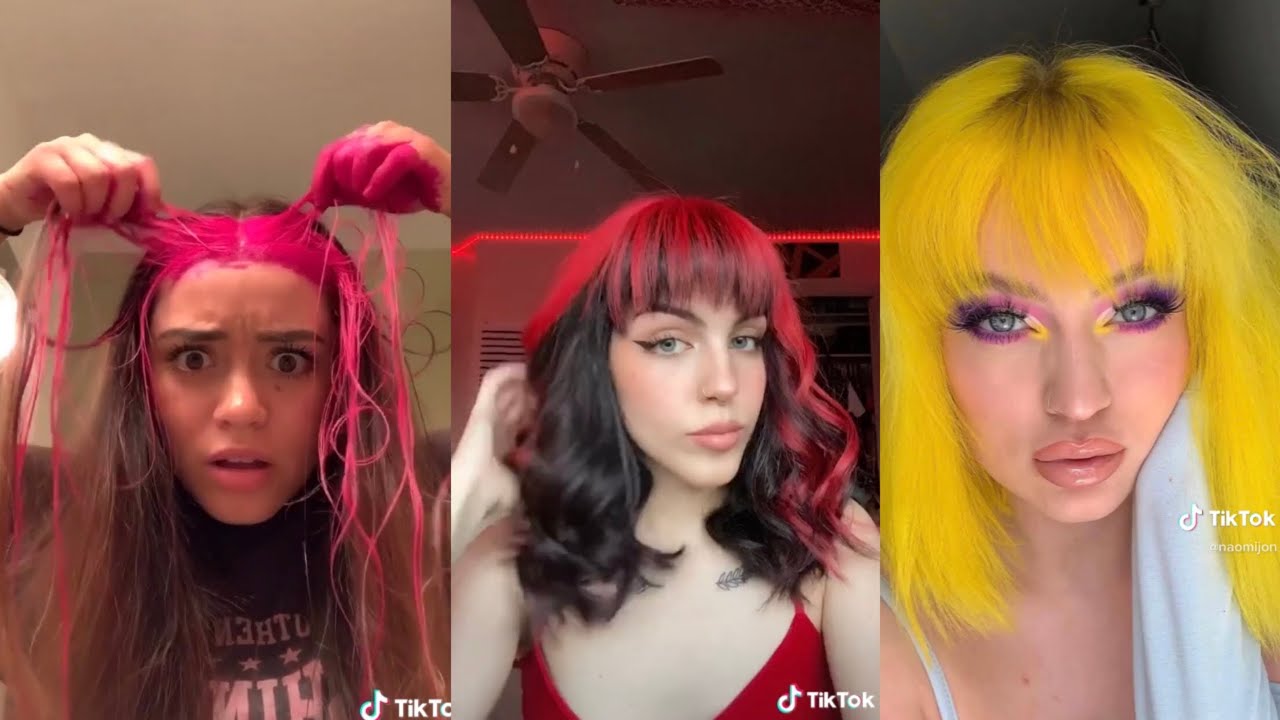This is a series of three images, each with the TikTok logo in the bottom right corner, showcasing three women with distinctive hair and makeup styles. On the left, a woman with brown hair has attempted to dye the front strands a vivid, hot pink hue. Holding up the strands with both hands, her right hand also streaked with dye, she wears a black t-shirt and displays a shocked and distraught expression, indicating her dissatisfaction with the outcome.

In the middle image, another woman is seen in a low-cut red spaghetti-strap top. Her shoulder-length, wavy hair features red streaks in the bangs and down the sides, set against a backdrop illuminated by pink LED lights, adding to the vibrant atmosphere. 

The woman on the right has all her shoulder-length hair dyed a striking yellow, complemented by heavy makeup with false lashes. Her eye makeup includes pink mascara or eyeshadow and yellow eyeshadow at the inner tips of her eyes, paired with a heavy nude lipstick. She wears a white spaghetti-strap top and has a composed, professional influencer appearance. Despite their varied looks, all three women stand out with their bold and expressive styles.